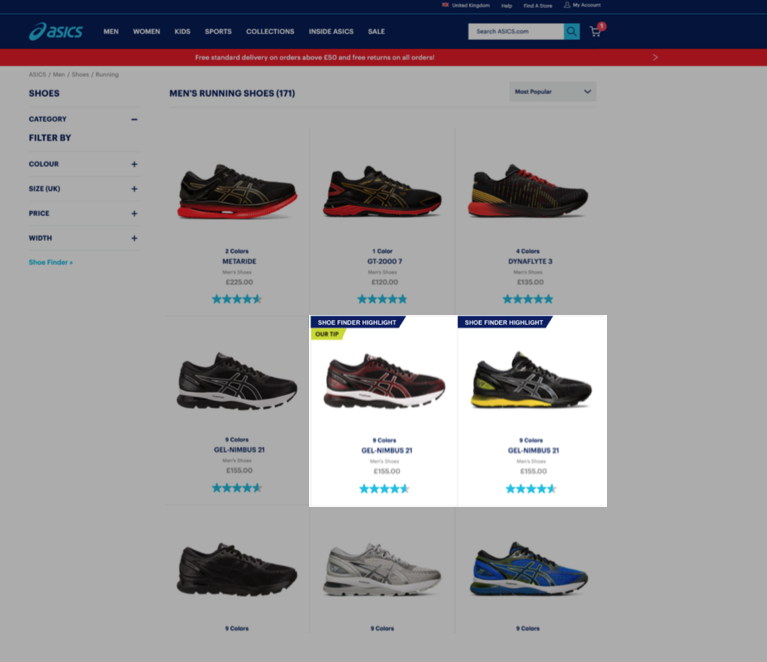This detailed vertical image captures the interface of a website, likely intended for viewing on a computer or smartphone. At the top, a horizontal rectangular blue banner dominantly displays the text "A6" in a distinct blue font. Below it, navigation categories such as Men, Women, Kids, Sports, Collections, Inside A6, and Sale are clearly listed. Adjacent to these options is a search bar and a shopping cart icon indicating one item. Above this navigation bar are utility options including United Kingdom, Help, Find a Store, and My Account.

Beneath the navigation, a red strip pronounces a promotional message stating "Free standard delivery on orders above £50 and free return on all orders," although the text is slightly out of focus. 

On the left-hand side of the image, there is a filter menu allowing users to refine their search by categories such as Shoes, Color, Size (noted as UK sizes in parentheses), Price, Width, and Shoe Finder. The main body of the interface is subtly grayed out due to a central white pop-up box that obscures part of the screen. Despite this, it is visible that the grayed-out background displays a selection sorted by most popular men's running shoes, complete with star ratings, names, and prices.

The white pop-up box titled "Shoe Finder Highlight" contains two shoe options under "Our Tip," showcasing them prominently to guide user decisions.